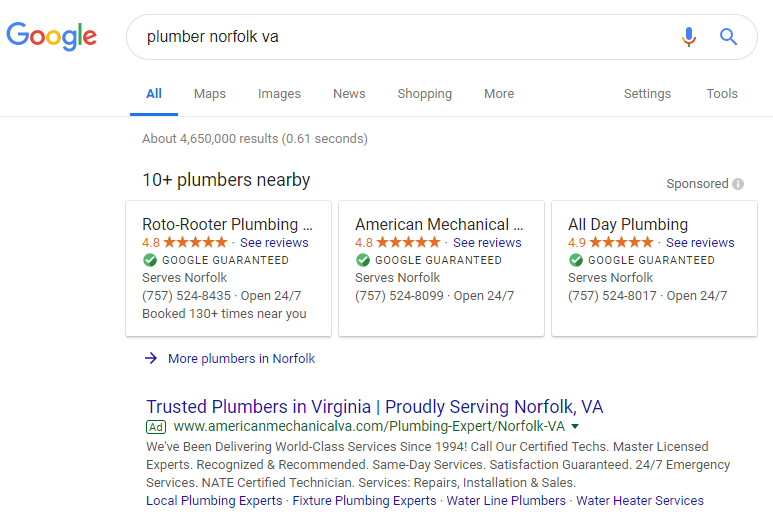Here's a detailed and cleaned-up caption for the image described:

---

This image depicts Google's homepage. The majority of the background is white. At the top center of the page is the iconic Google logo, with letters colored in the order of blue, red, yellow, blue, green, and red. Directly below the logo is a large search bar stretching across to the right. Inside the search bar, in black lettering, the text reads "plumber Norfolk VA." To the right of the search bar are a blue magnifying glass icon for search and a blue microphone icon for voice search.

Below the search bar are navigational options. From left to right, they are: "All" (underlined in blue), then "Maps" in black, "Images," "News," "Shopping," and "More." "Settings" and "Tools" are placed towards the right with a small space separating these from the other options.

Underneath this navigation bar, the search results begin. The text indicates that there are search results displayed along with the time it took to generate them. The first section of results is labeled "Sponsored" and contains three squares, each featuring different plumbers' information. Each square includes:
- The plumber's name
- Customer ratings and the number of reviews
- A green Google Guaranteed checkmark
- Service areas and phone numbers
- Business hours

To the right of these squares, a blue arrow points to the right with the text "More plumbers in Norfolk" next to it.

Further down, a larger link in blue text reads "Trusted plumbers in Virginia." A vertical line separates this text from additional information that reads:
"Proudly serving Norfolk, VA." Below this, the label "Ad" is displayed within a green square, with accompanying text and an email address. Finally, there are four lines of additional information about the advertisements.

---

This caption provides a comprehensive and vivid description of the Google search results page as detailed in the voice description.